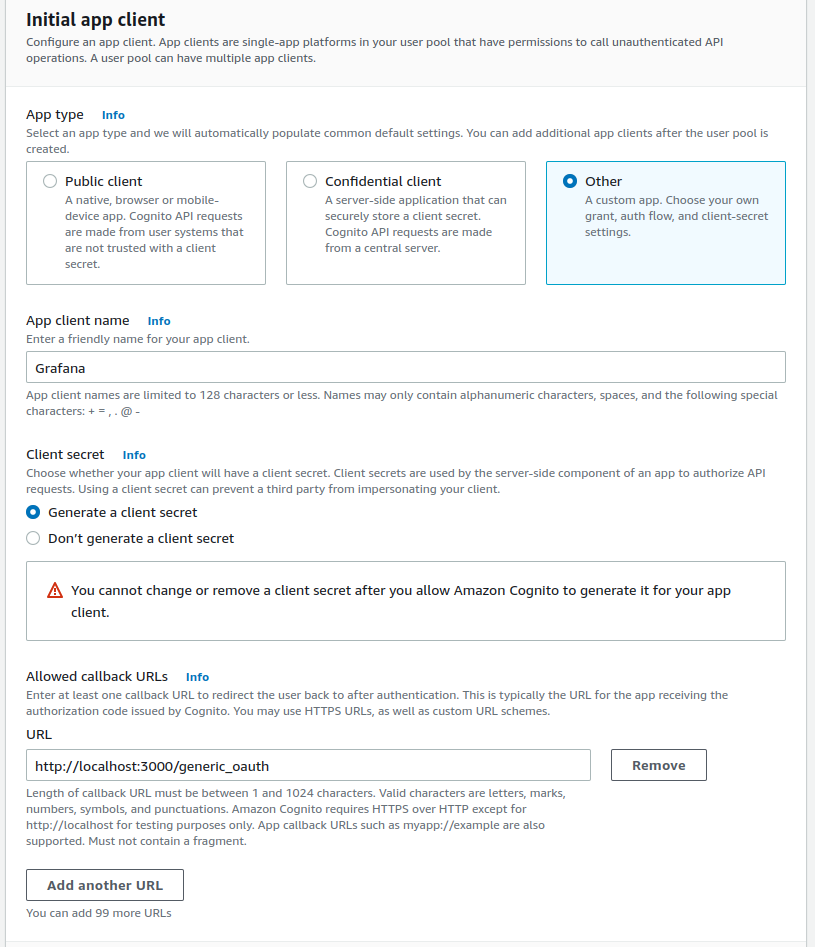Title: Detailed Information Sheet for Configuring an App Client in Amazon Cognito

Description: A detailed information sheet provides instructions on how to configure an app client in Amazon Cognito. The document is set against a white background and encompasses various sections with specific guidelines and options for setting up an app client. The key content includes:

1. **Initial App Client Setup**:
   - **Title**: "Initial App Client"
   - **Subtitle**: "Configure an App Client"
   - **Description**: "App clients are single app platforms in your user pool that have permissions to call unauthenticated API operations. A user pool can have multiple app clients."

2. **App Type Information**:
   - **Title**: "App Type Info"
   - **Description**: "Select an app type, and we will automatically populate common default settings. You can add additional app clients after the user pool is created."
   - **Options**:
     - **Public Client**: A native, browser, or mobile device where Cognito API requests are made to systems that are not trusted with the client secret.
	   - **Confidential Client**: A server-side application that secures and stores a client secret, where Cognito API requests are made from a central server.
	   - **Other**: A custom app, where specific grant authentication methods and client secret settings are chosen individually.
   - **Current Selection**: "Other"

3. **App Client Details**:
   - **Title**: "App Client Details"
   - **Fields and Options**:
     - **App Client Name**: Instruction to "Enter a friendly name for your app client." Example Name: "Grafana"
     - **Client Secret**: Option to generate or not generate a client secret. In this case, "Generate" is selected.
     - **Description**: "Client secrets are used on the server-side component of an app to authorize API requests. Using a client secret helps prevent third parties from impersonating your client. Note that once generated, the client secret cannot be changed or removed."

4. **Allowed Callback URLs**:
   - **Title**: "Allowed Callback URLs"
   - **Instruction**: "Enter at least one callback URL to redirect the user back to after authentication. This is typically the URL for the app receiving the authorization code issued by Cognito."
   - **Example URL**: "http://localhost:3000/genericOAuth"
   - **Options**:
     - **Remove Button**: To remove an existing URL.
     - **Add Another URL Button**: To add additional callback URLs.

Overall, the information sheet is a comprehensive guide for users to correctly configure their app clients, with a clear emphasis on securing API requests and managing authentication redirections.